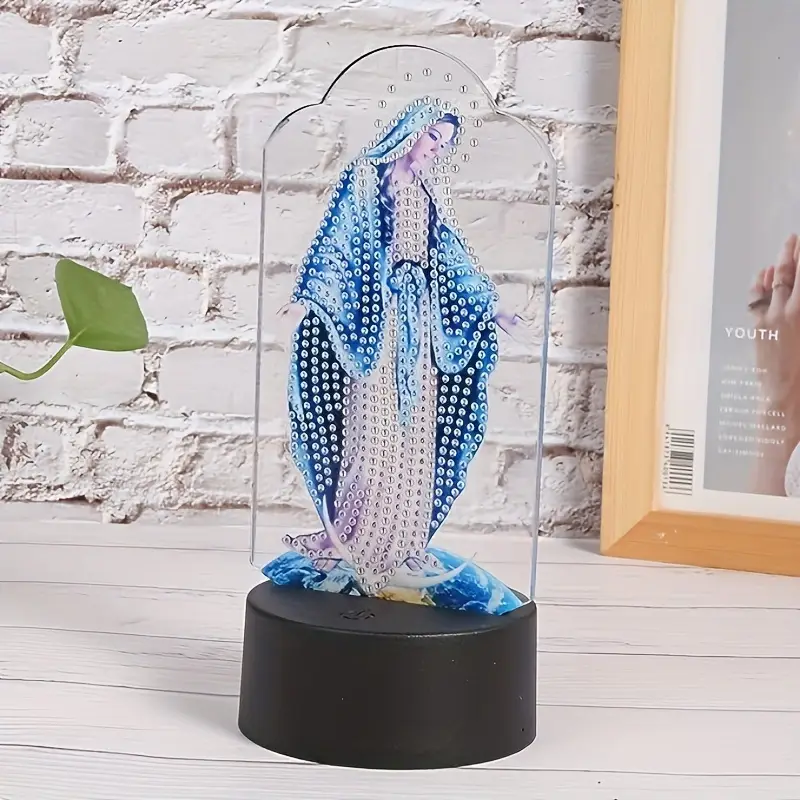The image depicts a statue of the Virgin Mary encased in a glass or plexiglass dome-like cover, mounted on a black base that is about the size and thickness of a hockey puck. Mary is adorned in a striking outfit, featuring a white robe underneath a blue cape and veil, which is patterned with white dots resembling stars or small diamonds. The blue cloak graciously drapes over her shoulders and pools at her feet, with a blue waist tie accentuating her figure. The entire statue is situated on a white wooden surface, with a brick wall in the background. Additionally, there is mention of a leaf partially visible from the left center of the image and a framed picture with a brown border to the side. Despite some details suggesting it might be a clock due to the layout above, the primary focus remains on the detailed and serene depiction of the Virgin Mary.